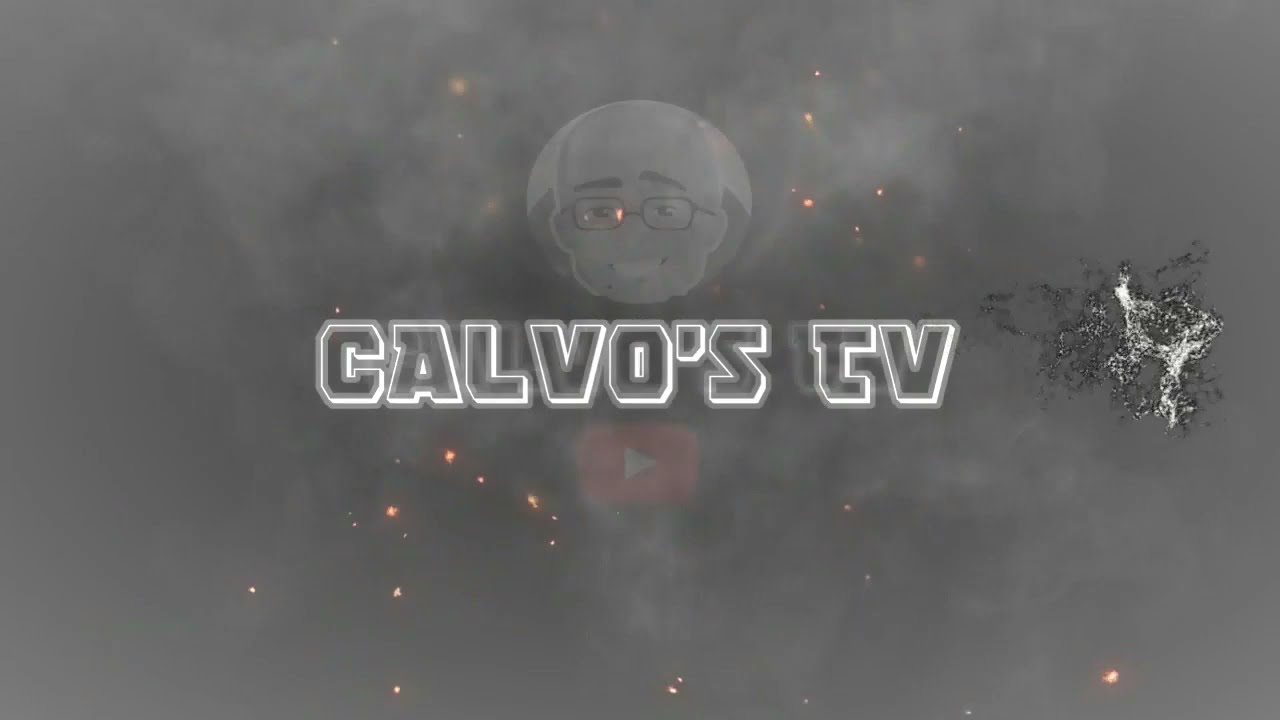The image has a predominantly gray background with a space theme, partly obscured by gray clouds or a smoky effect. There are hints of sparkles, possibly gold or orange stars, scattered throughout. Centered on the image, there's a circular, cartoon-like avatar of a bald man with black glasses and a wide smile, raising one eyebrow—the presumed "Calvo." Across the center of the image is the bold, all-caps text "CALVO'S TV" outlined in white. Below this text, there is a faint, iconic red YouTube play button, a red rectangle with a white triangle pointing right. To the right of the text, there's a black and white smear or ink blot, potentially representing an asteroid or another cosmic object.